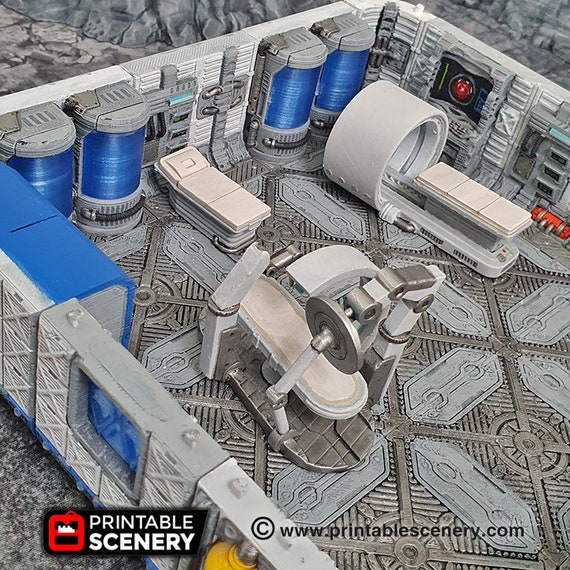The image depicts a detailed, resin-printed model of a futuristic medical facility, often referred to as a "moon base medical lab" from www.printablescenery.com. The scene includes modular components resembling high-tech medical equipment and environments, such as a patient cot, a radiology device, and vertical blue chambers. Notably, there is a white cylindrical structure with a red button, giving the appearance of advanced medical scanning technology. The setting, with its space-themed floor, suggests an extraterrestrial locale similar to a medical bay in a sci-fi universe, potentially echoing something from Star Trek.